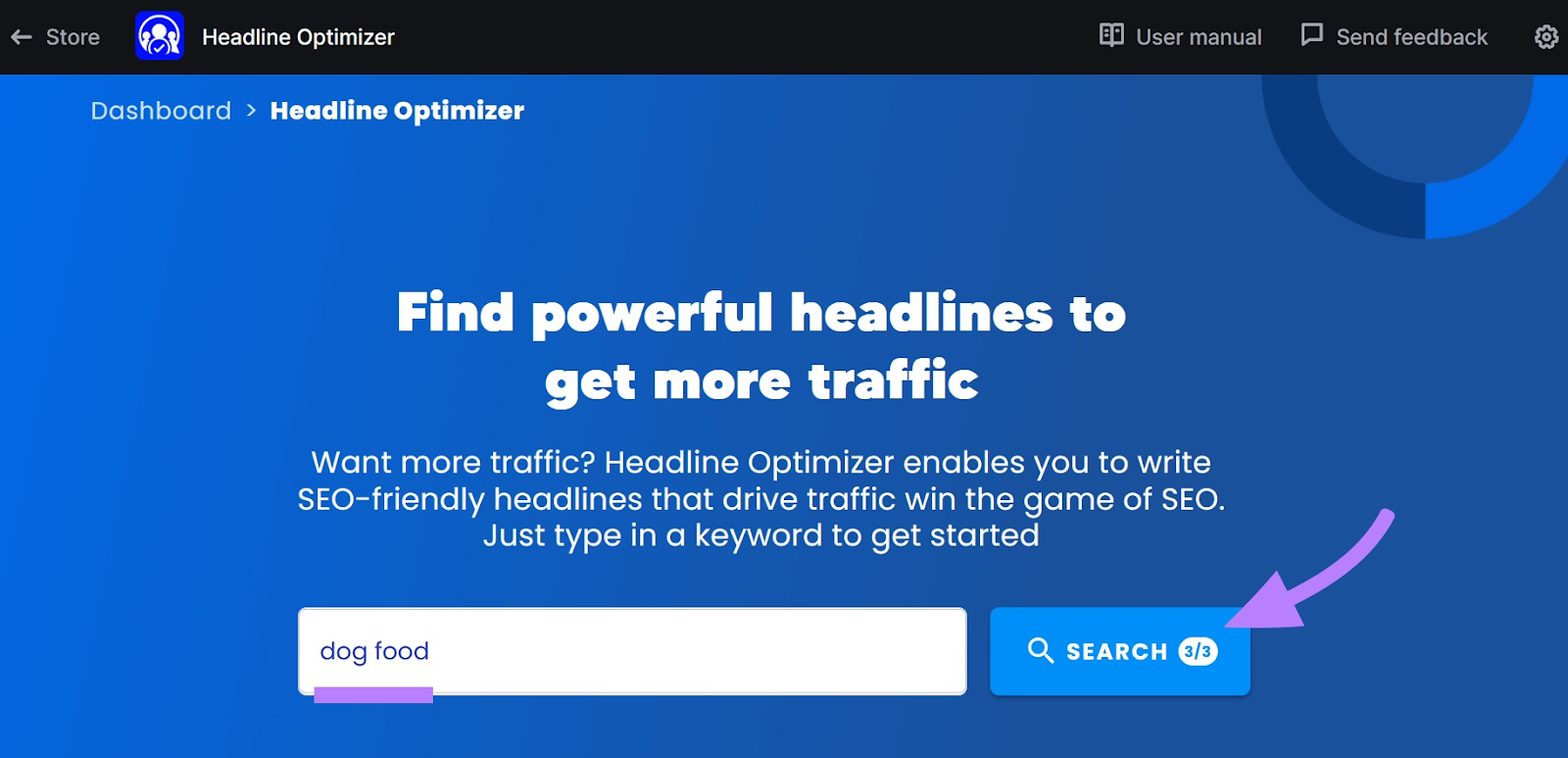The image showcases a visually structured interface, predominantly featuring a wide rectangle that is significantly broader than its height. The background is primarily blue, accentuated by a narrow black border at the top. 

In the top left corner, there's a small left-pointing arrow accompanied by the word "Store." Centrally aligned at the top, the bold white text reads "Headline Optimizer." On the top right, there is an icon of an open book labeled "User Manual." Adjacent to it, a speech bubble with the phrase "Send Feedback" appears next to a small gear icon.

Below this header section, the blue background continues. On the left side, the word "Dashboard" is displayed next to a small arrow, with "Headline Optimizer" prominently written in bold white text. Centered prominently in the middle of the page, the largest text on the image declares in bold white, "Find powerful headlines to get more traffic." 

Further below, in smaller white text, the caption reads: "Want more traffic? Headline Optimizer enables you to write SEO-friendly headlines that drive traffic and win the game of SEO. Just type in a keyword to get started." 

Below this description, on the left side, there's a text input box with a white background, containing the phrase "Dog Food" underscored by a thick purple line. On the right, a blue rectangle displays a white magnifying glass icon followed by the word "SEARCH" in all capitals. Below this, it reads "3/3," and a large purple arrow points towards this search box.